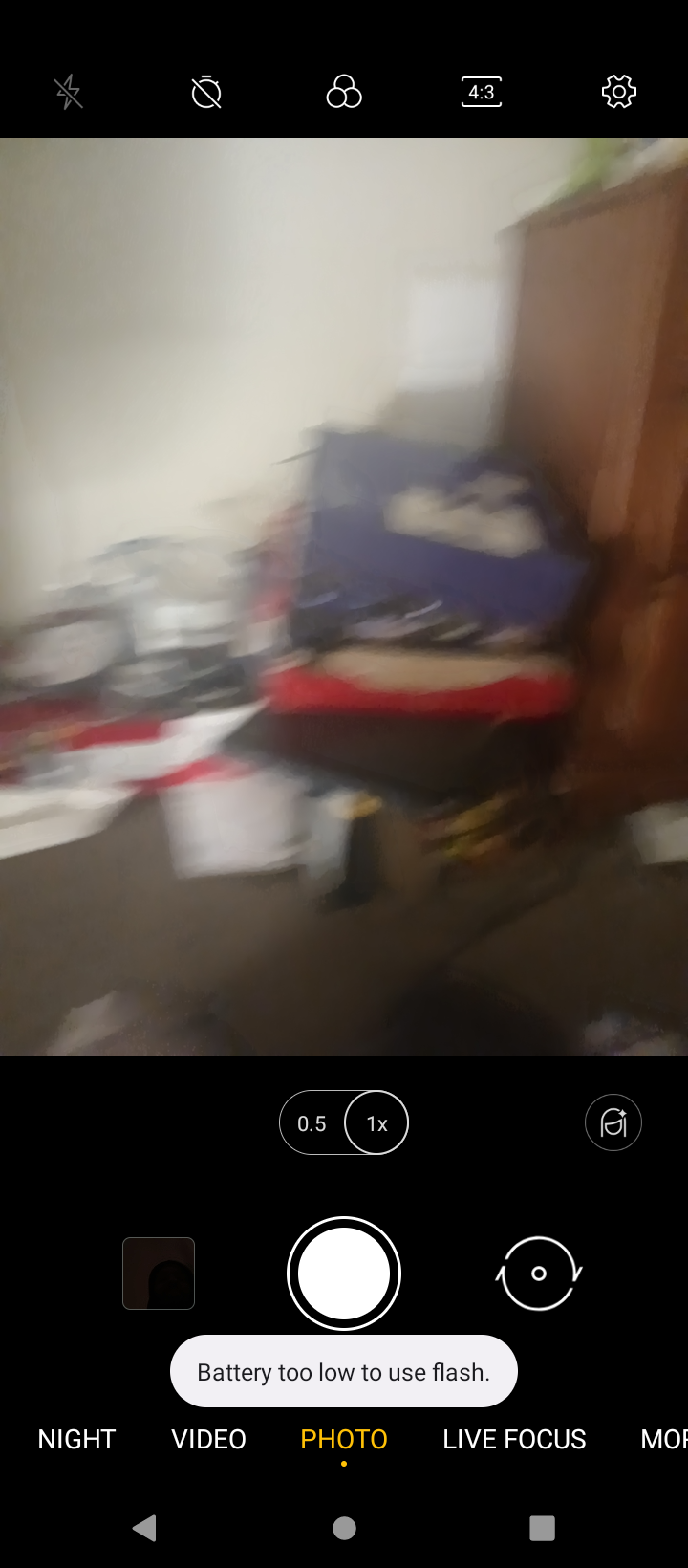This image is a screenshot of a camera application interface actively being used to photograph a cluttered room. The screen is framed by black bars at the top and bottom. At the top, the black bar features various white icons, including symbols for flash, settings (gear symbol), and other camera-related functionalities. Dominating the bottom black bar is a large, white circular button, commonly used for taking photos. Beneath this button, there is a white-text-on-black notification reading, "Battery too low to use flash," indicating the current low battery status of the device. The yellow word "Photo" is prominently displayed at the bottom, surrounded by additional white text options like "Night," "Video," "Live," and "Focus," suggesting different modes and features of the camera app. The camera is aimed at a disorganized, messy room, capturing piles of various items in a blurry, chaotic scene.